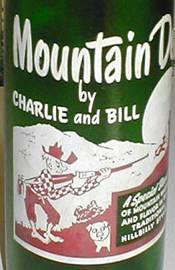The image features a close-up of a vintage, collector's edition Mountain Dew glass bottle, partially cropped to focus on the logo. Encased in green glass, the bottle displays a white and red screen-printed logo that prominently reads "Mountain Dew" by "Charlie and Bill," though the word "Dew" is partially obscured. The logo portrays a barefoot, plaid-clad, hat-wearing southerner holding a shotgun, seemingly aiming off-screen. Beside him stands a pig (or possibly a dog), contributing to the hillbilly motif. The southern character and his attire, along with the rustic setting, evoke a nostalgic, rural charm. A separate text box in the background, though partially out of frame, contains the word "Hillbilly." Overall, the image captures the essence of this old-fashioned Mountain Dew bottle with its distinct vintage design and screen-printed artwork.